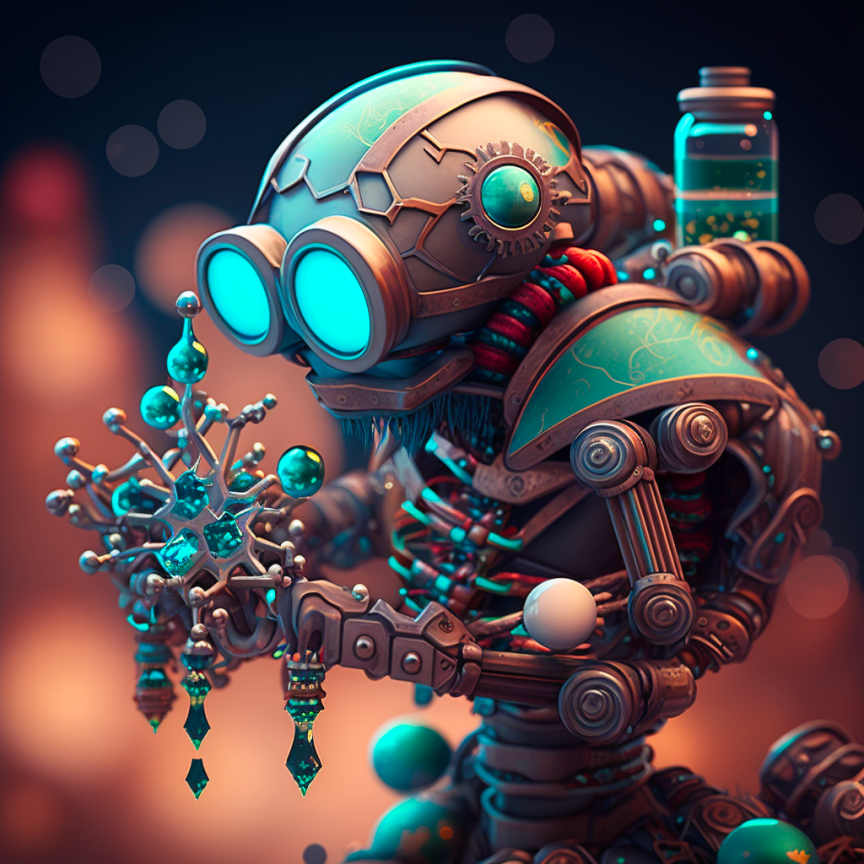This image features a meticulously detailed, AI-generated 3D rendering of a robot with a distinct steampunk aesthetic. The robot's design incorporates a blend of turquoise and brass-colored metal, giving it a mechanical yet fantastical appearance. It has large, glowing turquoise eyes reminiscent of steampunk goggles, which add to its unique charm. The robot’s upper body, including its shoulder pads and helmet-like headpiece, showcases a combination of teal and copper hues. One of the robot's striking features is its appendage that resembles a mechanical arm adorned with gems, extending outwards and ending in bulb-like structures. The overall impression of the image is that it resembles high-quality fan art, capturing a fusion of futuristic AI design and classic steampunk elements.